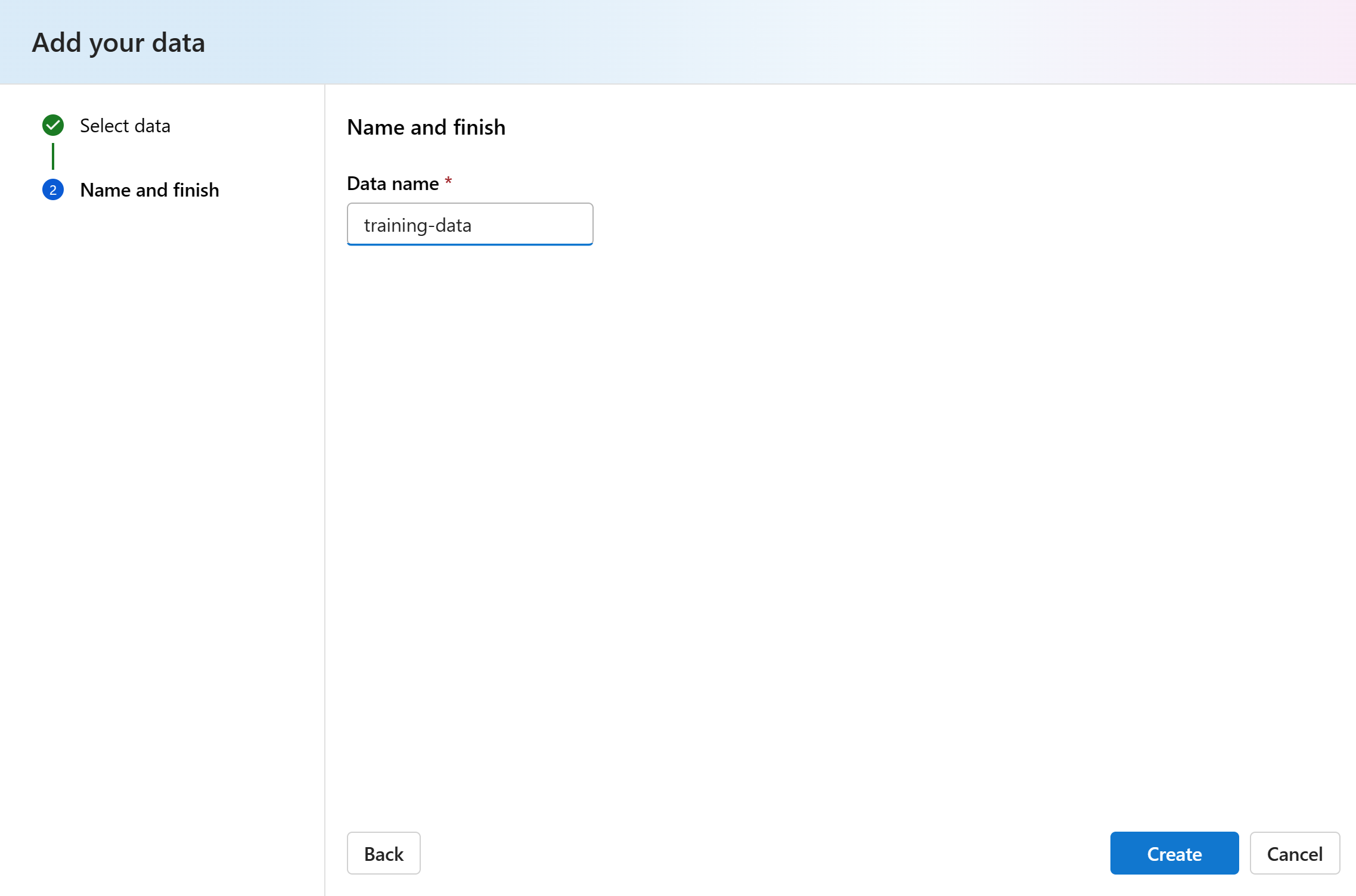This screenshot is from Microsoft Azure AI Studio. The top section of the interface prominently displays a header with the text "Add Your Data" on a light blue background that gradually transitions to a light purple towards the right. 

In the left pane, under the section labeled "Select Data," there is a green checkmark indicating completion. A vertical line extends downward from the green checkmark, connecting to a blue bubble numbered "2." Adjacent to this, the text "Name and Finish" designates the next step in the process.

The right pane is straightforward, featuring two main lines of text and interactive elements. The first line repeats "Name and Finish," while the second line prompts for a "Data Name," marked by a red asterisk to indicate a required field. A small input bar beneath this prompt has the text "training-data" pre-filled.

The rest of the screen is largely blank, with a white background dominating both the left and right panes. At the bottom-left corner, there is a "Back" button, and at the bottom-right corner, two adjacent buttons labeled "Create" (colored blue) and "Cancel."

The overall design is clean and minimalistic, with the left and right pane backgrounds in white, while the header distinctly stands out with its gradient effect from light blue to light purple.